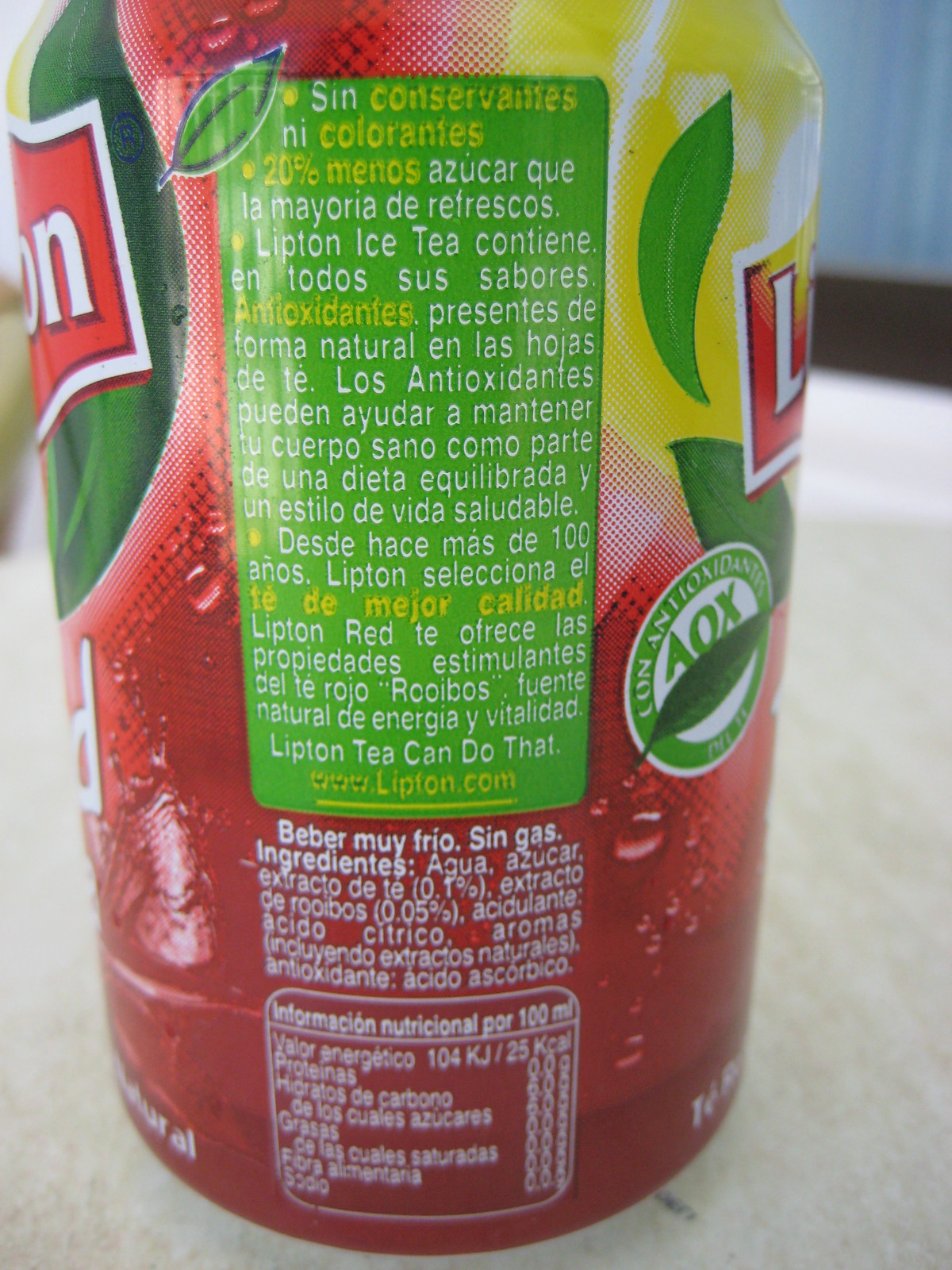This detailed, up-close photo showcases a 12-ounce can of Lipton iced tea with predominantly red coloring on an aluminum surface. The can prominently features Lipton’s logo, which is red and white, with a green rectangle positioned centrally on the label. This green section provides nutritional information and ingredients, mostly written in white and yellow text. Although the majority of the can’s labeling is in Spanish, key points detailed include "sin conservantes ni colorantes" (indicating no preservatives or artificial coloring) and a claim of 20% less sugar than typical sugary beverages. The website www.lipton.com is also visible on the label, identifying this as a healthier variant of Lipton iced tea. The photograph is captured in portrait orientation, focusing closely on the intricate details of the can, including the ingredients and nutritional facts displayed toward the bottom.